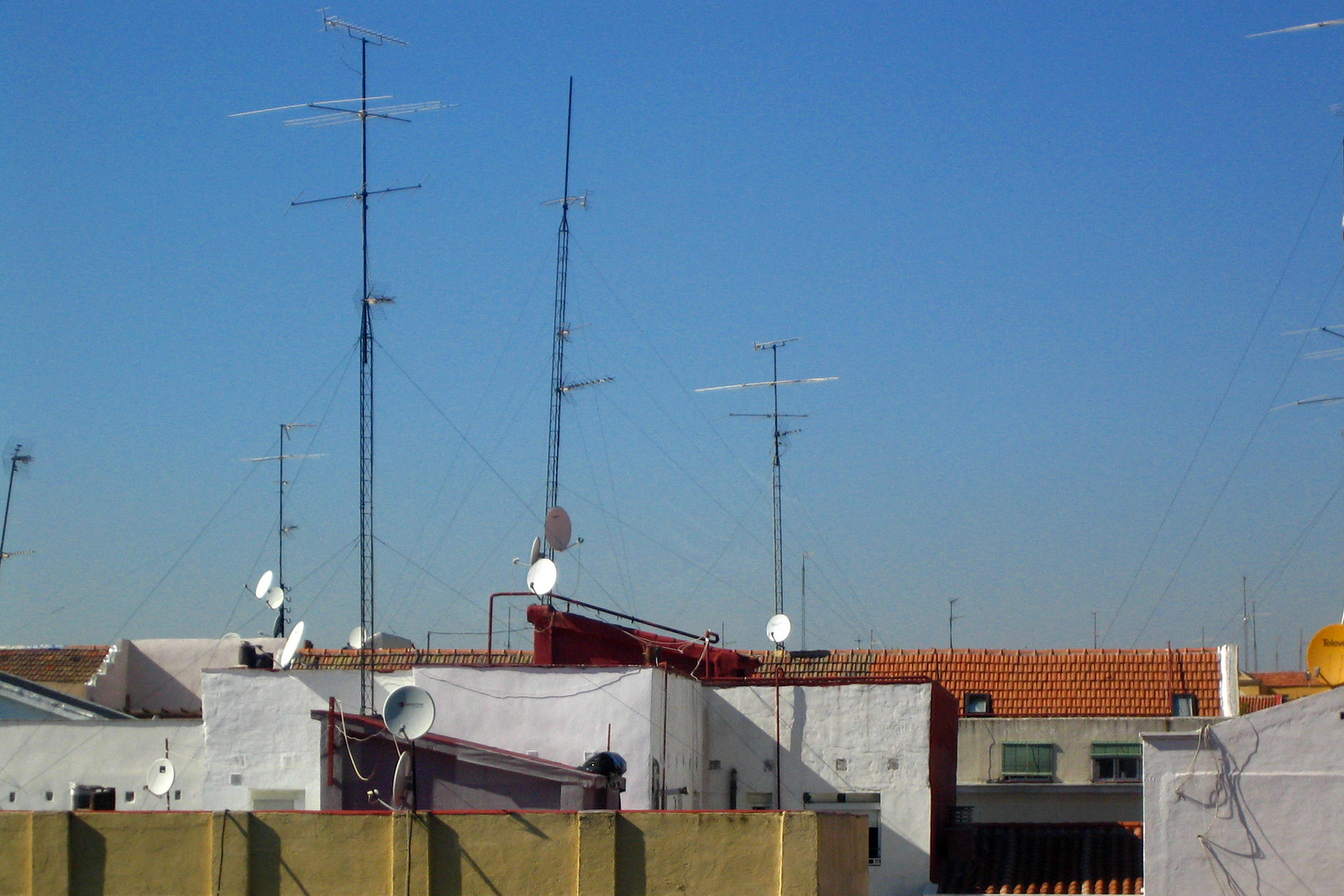This detailed photo captures a cluster of urban rooftops with varied features. Dominating the scene are several buildings: a white cement building with a red-tiled roof, a yellow brick building with white satellite dishes, and a gray building in the vicinity. The rooftops, particularly of the white building, display an array of satellite dishes—one building sports four on its red roof. Notably, there's an orange tiled roof visible further back. Rising prominently into the clear blue sky above these structures are large radio towers, characterized by their metal scaffolding and crossbars, topped with multiple parallel metal rods forming a radio array. Additional elements like windows, various roof tiles, and attached wires add to the intricate details of the urban landscape. The sky, a gradient from clear blue at the top to a grayer hue nearer the horizon, forms a stark backdrop to the bustling array of antennae and satellite dishes.